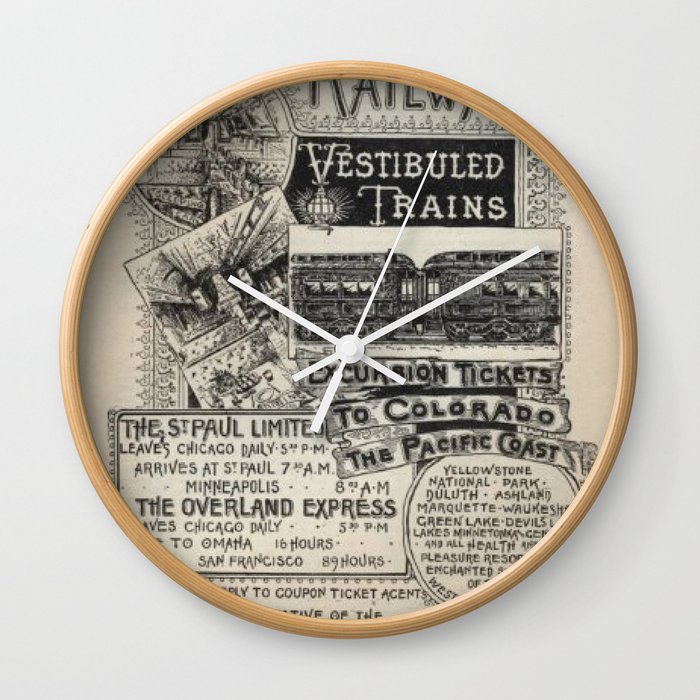This photograph captures a uniquely designed clock with a light wooden circular frame. The clock’s face is devoid of traditional numerals and instead features a meticulously detailed graphic focusing on train memorabilia. At the top, a black rectangle with white text reads "Vestibule Trains," accompanied by a charcoal-style drawing that illustrates the junction of two train compartments. Below this are white strips with black text that advertise "Excursion tickets to Colorado, the Pacific Coast." Further down, a circular white background displays place names such as "Yellowstone National Park, Duluth, Ashland, Marquette, Waukesh, Green Lake, Devils Lake, Minnetonka" alongside phrases like "All Health, Pleasure, Enchanted," although some text is obscured by the frame. To the left, additional text on a white background provides details of train schedules: "The St. Paul Limited leaves Chicago daily, 5.30pm arrives at St. Paul, 7.30am, Minneapolis, 8am. The Overland Express leaves Chicago daily, 5.30pm, to Omaha, 16 hours, San Francisco, 89 hours." The clock features white hands indicating the second hand at approximately 1 o'clock, the minute hand at about 2 o'clock, and the hour hand at approximately 10 o'clock. The entire design, rendered in black and white with a papyrus-like background, suggests this clock is a collector’s item, framing historic train travel graphics and schedules, encased within its timeless wooden border.